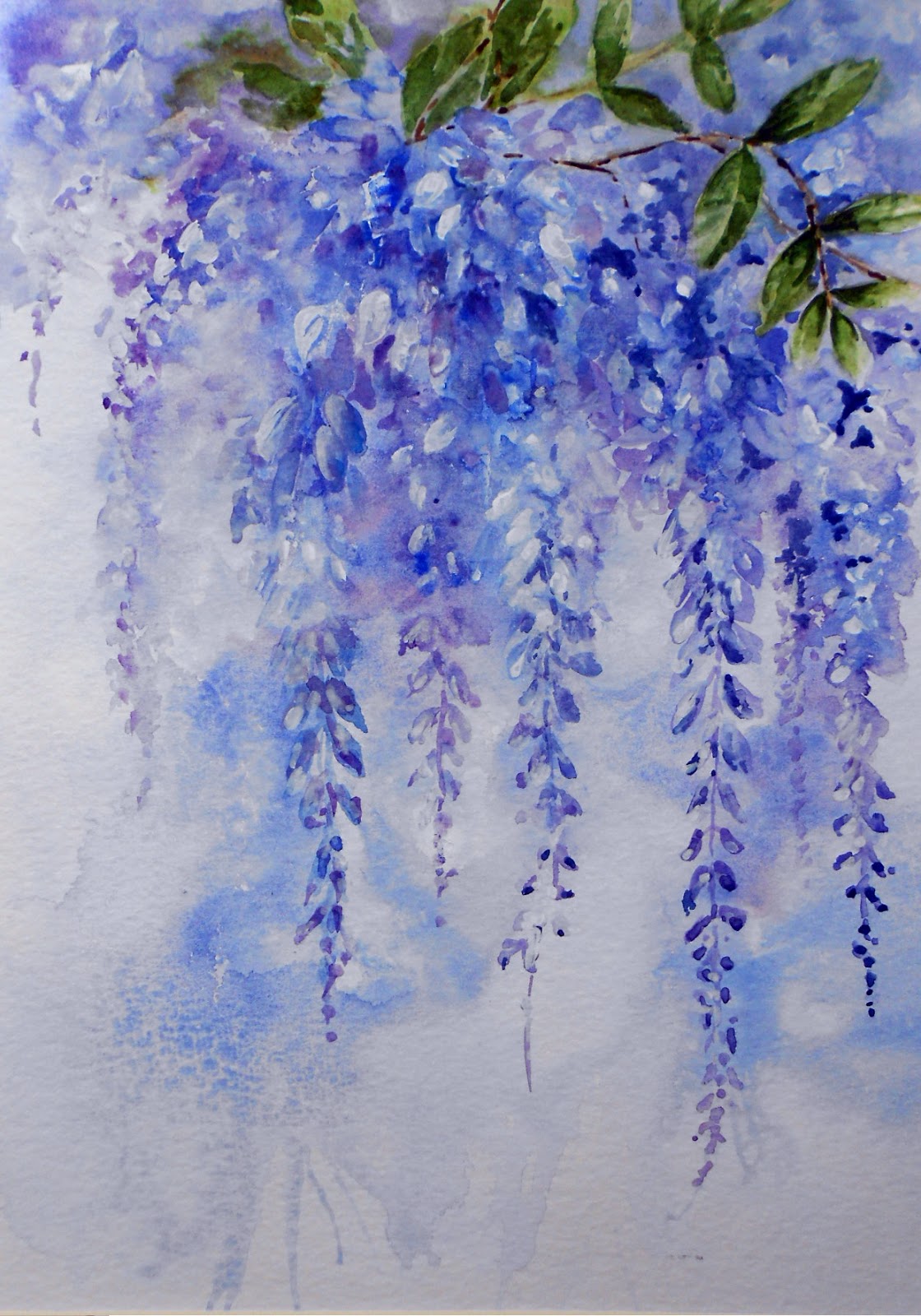This watercolor painting captures an impressionistic, almost ethereal depiction of a delicate flowering plant. Dominated by a palette of blue shading into purple, the image features a sprig of woody material at the top with feather-shaped green leaves and small branches. Below this is a dramatic cascade of flowers that drape down across approximately 80 percent of the page. These flowers, painted in varying shades of blue, purple, and white, dangle like delicate, iced-over tendrils, each with a defined appearance, almost resembling octopus legs. The background is a blend of white and off-white with subtle blue watercolor accents, enhancing the delicate and slightly blurry essence of the flowers. The overall impression is one of vibrant yet gentle beauty, capturing the intricate yet softened details of the flowering plant.